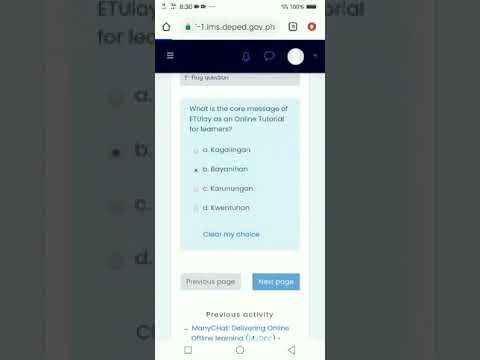This image is a blurred and somewhat small screenshot from an Android phone, displaying a web page in Google Chrome. The webpage appears to be part of an online tutorial or quiz, with a light blue background and a multiple-choice question asking, "What is the core message of Thule as an online tutorial for learners?" Below the question are four different answer choices and an option to clear the selection. The navigation includes a grey "Previous page" button and a blue "Next page" button. Additional text mentions a "previous activity" and other options like "Many chat" as well as "delivering online, offline learning". The phone's status bar is visible, showing the number of open tabs, the address bar, and the remaining battery power. The overall layout shows sections on the left and right, but they are largely obscured and fragmented.